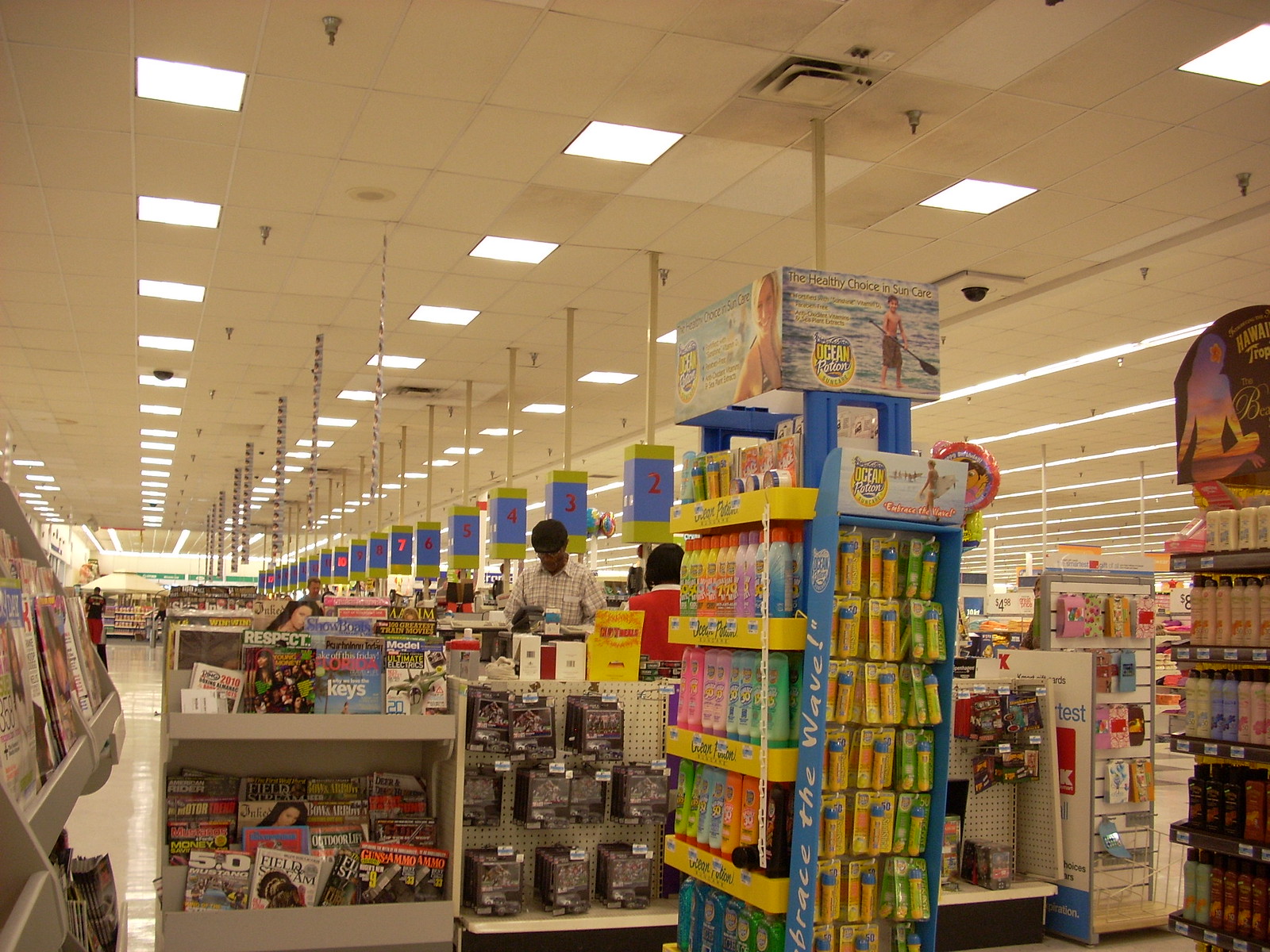The image captures the bustling interior of a large grocery store's checkout area. Lined with numbered lanes ranging from 1 to about 20, each checkout is marked by blue and yellow light boxes displaying their respective numbers, with some illuminated such as number 7. Customers, like a young man in a white checkered shirt, navigate the aisles assisted by attendants in red vests. The foreground features a white shelf adorned with an array of colorful magazines, their positions notably in the bottom left and middle sections. Adjacent to the magazine rack is a tall display of suntan and sunscreen products, showcasing an assortment of metal and plastic bottles in vibrant hues of green, pink, and blue. Nearby, another rack is dedicated to shampoos and a variety of hanging items. Overarching the scene, the white-tiled ceiling hosts neatly arranged square lights and sprinklers, from which poles extend to the blue light boxes, creating an organized, well-lit environment. The far left of the room transitions into produce sections, while other aisles extend along the right side, completing the comprehensive snapshot of this well-equipped shopping area.